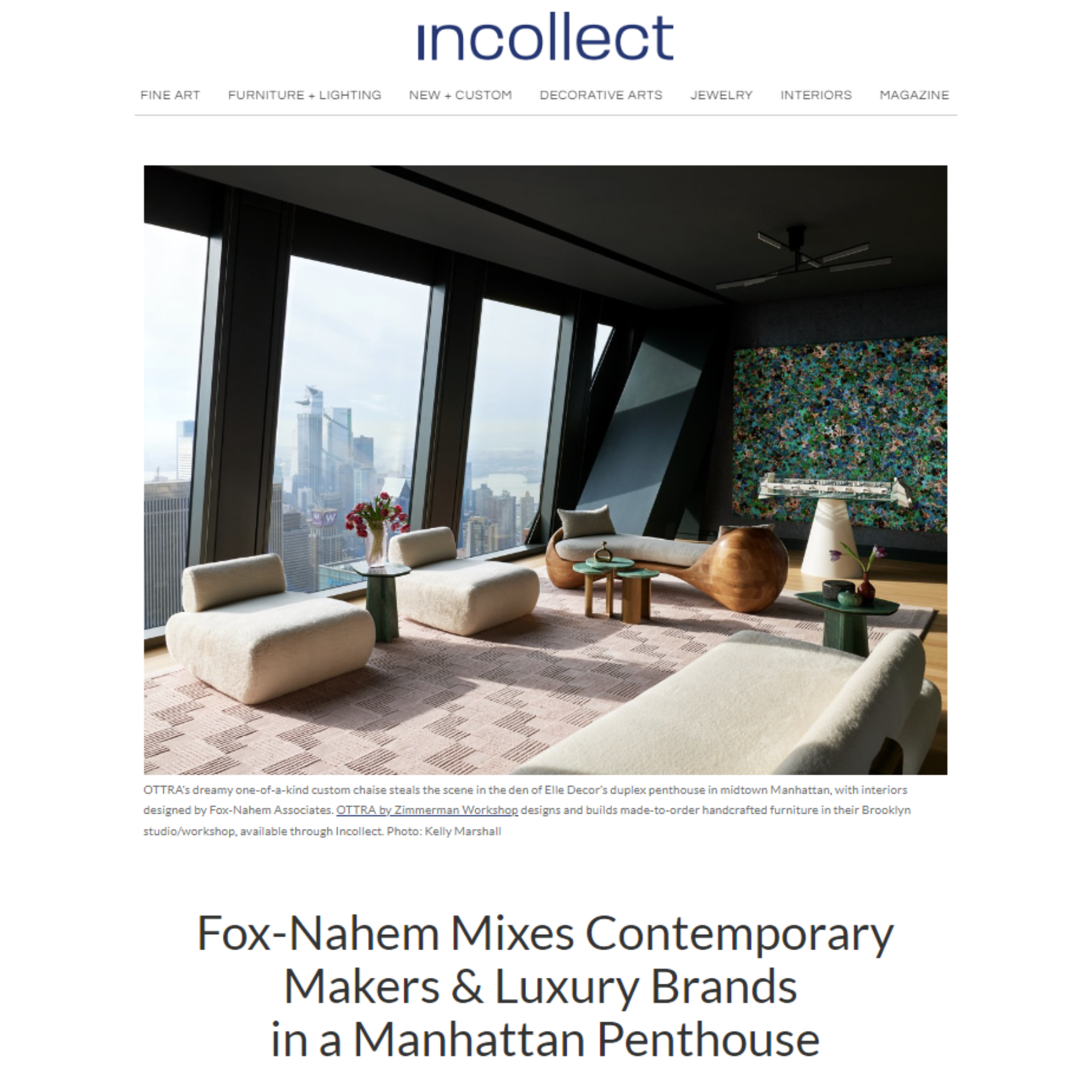The image is a magazine page with a clean, white background showcasing a website or advertisement. The header features the blue text "INCOLLECT" followed by a navigation bar listing categories such as Fine Art, Furniture and Lighting, New and Custom, Decorative Arts, Jewelry, Interiors, and Magazines. Below this, an opulent photograph captures a luxurious, well-decorated penthouse in Manhattan, designed by Fox Nahem Associates. The interior exudes sophistication with neutral tones, including beige couches and a light tan rug, complemented by various wood accents. The space boasts three large, rectangular windows offering a city skyline view, framed by dark green walls and a black ceiling. A striking artwork featuring greens, blues, and pinks adorns the background. Notable furnishings include a pair of light tan chairs, an end table with a plant, an upscale coffee table positioned between the seating arrangements, and a black ceiling fan. Beneath the image, the text highlights OTTRA's custom-made furniture, crafted in their Brooklyn studio and available through INCOLLECT, with a photo credited to Kelly Marshall. A prominent caption at the bottom reads, “Fox Nahem mixes contemporary makers and luxury brands in a Manhattan penthouse.”